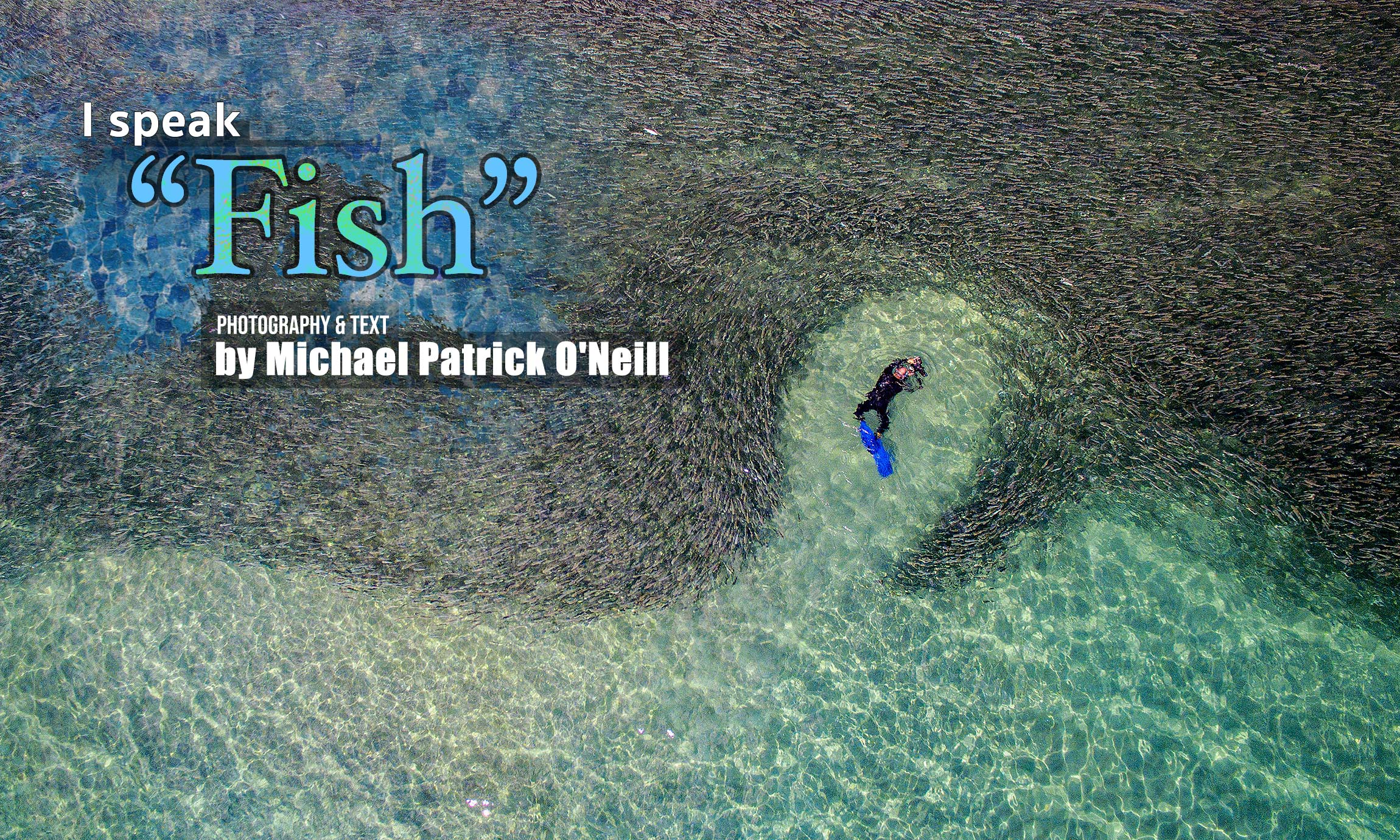This aerial photograph, captured and annotated by Michael Patrick O'Neill, depicts a diver immersed in a vast, shallow expanse of clear blue water, likely over a coral reef. The diver, clad in a black wetsuit and blue flippers, navigates through a dense shoal of fish that dynamically form patterns around him as he swims. Taken from above, the image also shows varying shades of the ocean, with darker areas indicating depth. The diver appears to be taking photographs of the fish, capturing the moment from below. The image includes the text "I speak 'fish'," emphasizing the diver's deep connection to the marine life.